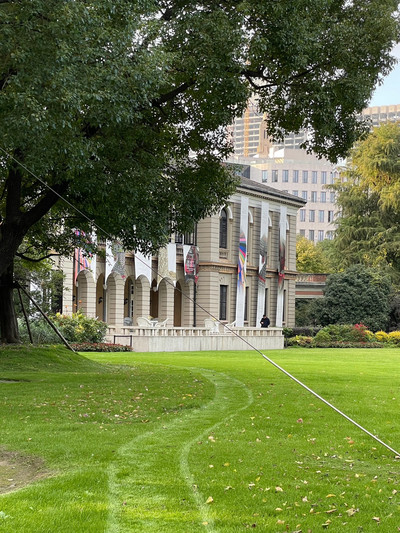A vibrant color photograph captures a picturesque scene of a stone building nestled behind a sprawling, green lawn. Tire tracks from a small vehicle mark the foreground of the lush grass. Dominating the left side of the image, a large tree extends its leafy branches, providing partial shade. The stone building features an elegant archway at its entrance, flanked by a robust stone wall. Lawn furniture, arranged for relaxation, adds a casual charm, while white banners adorned with indiscernible colored decorations hang from the building's front wall.

A man leans casually against the wall, absorbed in his cell phone. Surrounding the building, a thoughtfully designed landscape includes bushes with clusters of yellow flowers to the left and right. In the background, tall buildings and stately trees rise against a clear blue sky, just visible in the upper right-hand corner of the composition. This serene and inviting scene harmoniously combines elements of architecture, nature, and daily life.